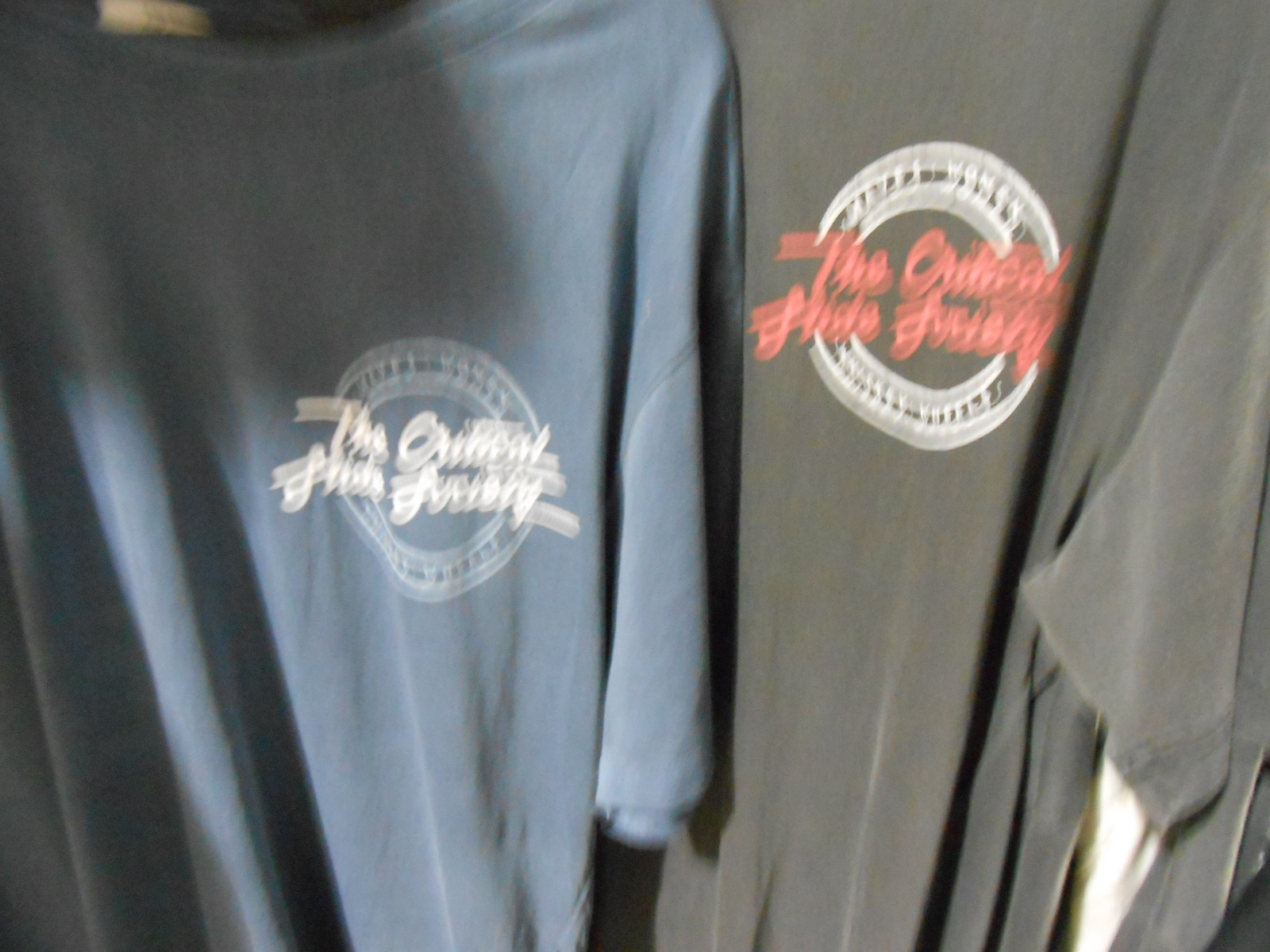The image depicts a slightly blurry photograph of two t-shirts placed next to each other horizontally. The t-shirt on the left is blue, featuring a logo on the upper right breast area. The logo comprises white cursive text, with a white circle beneath this text. Details within the circle are not clearly visible. On the right, the second t-shirt is a dark washed-out gray color and also displays a similar logo. This logo, however, consists of red cursive text set against a white circle background.